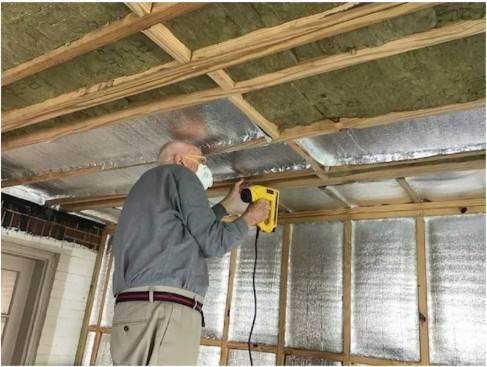This detailed color photograph captures an elderly man, approximately 70 years old, engaged in a home renovation project, possibly in a garage or a room under construction. The man, wearing an N95 respirator and safety glasses, is dressed in a long-sleeved gray shirt, khaki pants, and a black belt with a red stripe. He holds an electric stapler or nail gun, distinguished by its yellow color and attached black cord. The ceiling and walls are in the process of being insulated with shiny, silver insulation paper. Wooden beams and studs are visible around the room, indicating a work-in-progress. A gray door stands to the far left, and a section of the room's structure features bricks.